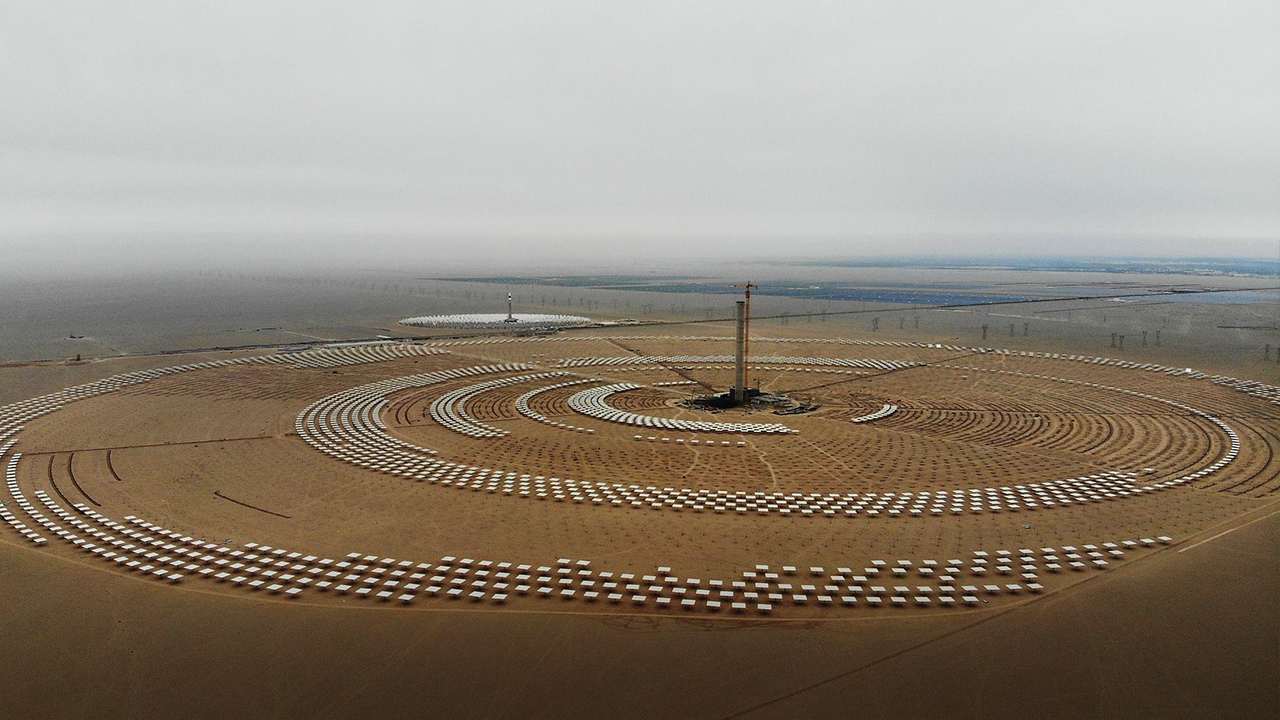The image depicts a vast, flat landscape that appears to be made of sand or dirt, leading to a foggy, overcast sky. There are some large water bodies, such as lakes or ponds, situated in the background. Spread out in a circular and spiral pattern across the lower portion of the image are arrays of raised white platforms or tiles, evenly spaced and mounted on posts. These structures create concentric circles that incrementally move inward towards the center of the image. In the very center, there are two large vertical posts—one possibly made of concrete and the other of metal—encircled by a clear, minimally marked area. The arrangement suggests a manmade, possibly industrial or research-based setup, etched into the grooved dirt of this expansive field.